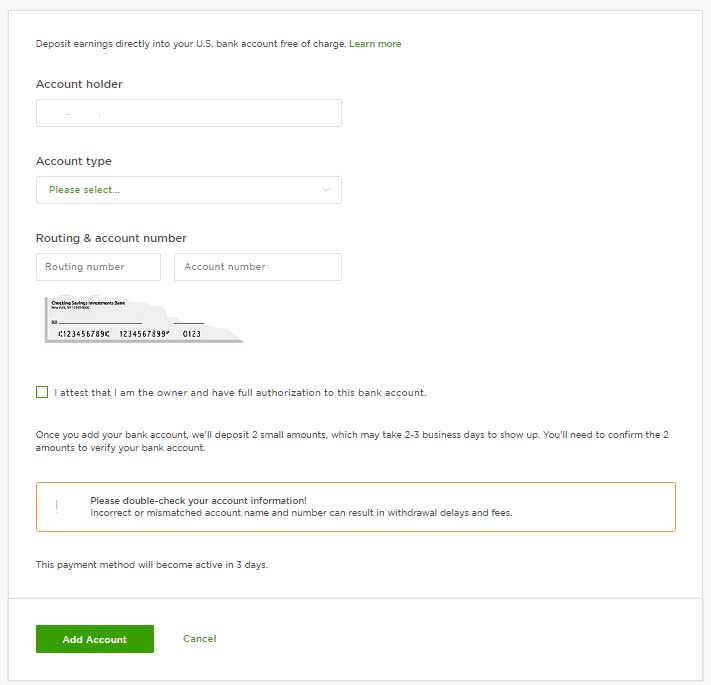The image depicts a form for directly depositing earnings into a U.S. bank account, free of charge. The form includes fields for the account holder's name, routing number, and account number. There is a checkbox that needs to be marked to confirm that the bank account does not belong to an organization. Once the bank account information is added, two small deposit amounts will be sent to the account, which may take up to two or three business days. The form instructs the user to confirm these amounts, which will activate the payment method in three days within the account. Users are advised to double-check their account information to avoid incorrect matches, as errors could lead to withdrawal delays or fees.